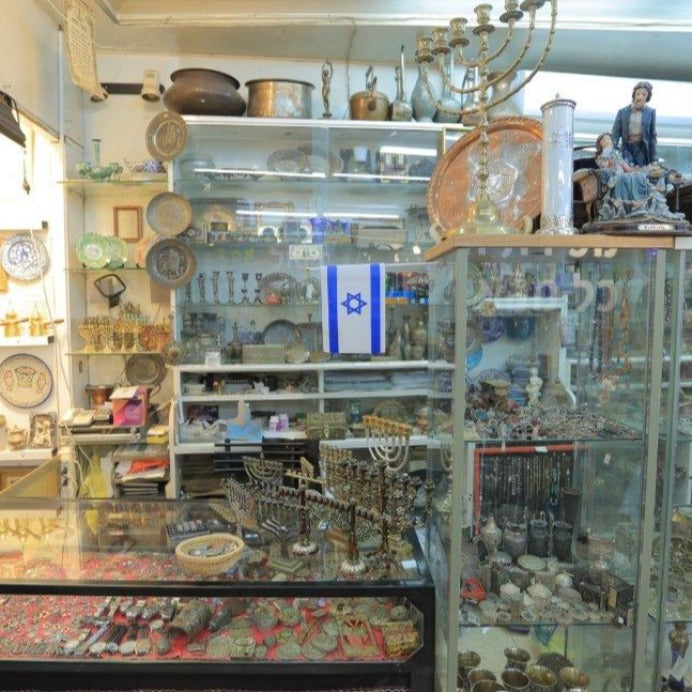The image depicts the inside of a densely packed shop brimming with a diverse assortment of items, with a strong emphasis on Jewish antiques and memorabilia. The back wall and shelves behind a counter are adorned with multiple shelves that extend high up, displaying jewelry, various menorahs, and a flag of Israel. The glass cases in front of the counter are filled with a multitude of small items, including coins, brass work, necklaces, and jewelry. On top of these cases lie porcelain figurines and aluminum bowls. To the right, another glass cabinet showcases statues and more assorted memorabilia. The entire space is cluttered with an array of candles, silver plates, bowls, picture frames, and baskets, providing a visual feast of religious symbols and intricate artifacts, evidently all for sale.